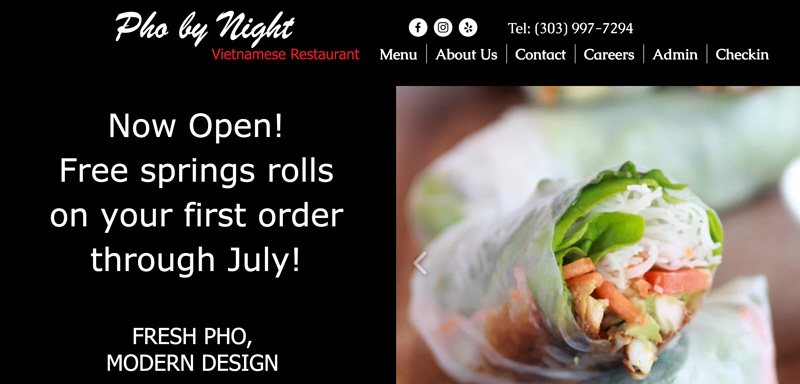This image showcases the header section of a Vietnamese restaurant's website menu. At the top, the restaurant name, "Pho By Nyg*ht," is prominently displayed in white, italic-like font against a dark background. The unique spelling of the name is clearly visible as "P-H-O space B-Y space N-Y-G-H-T." To the right of the restaurant name, a series of social media icons is neatly arranged: a Facebook circle icon, an Instagram circle icon, and another circle icon with an asterisk in the center. Each icon is white with the symbol in black.

Next to the icons, there is the restaurant's contact information, displayed as "TEL: 303-997-7294." Beneath "Pho By Nyg*ht," in red font, a line indicates that it is a Vietnamese restaurant. Further below on the right-hand side, a promotional text in red announces, "Now open. Free spring rolls on your first order through July." Adjacent to this text, on the extreme right, is an image of what appears to be a wrapped food item, potentially illustrating one of the restaurant's menu offerings.